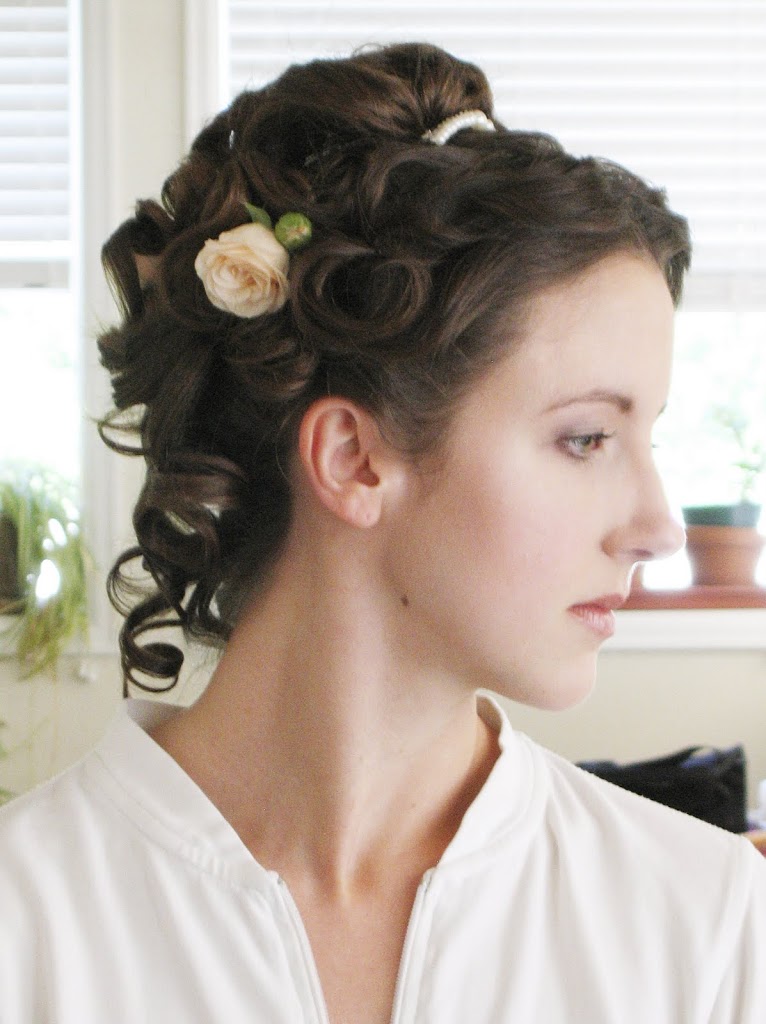The image features a close-up profile of a fair-skinned woman with dark brown hair elegantly styled in an intricate updo. Her body is facing towards the camera while her face turns over her right shoulder, her gaze directed downwards. The updo is detailed with several curls intricately clasped at the top with a pearl clip. A distinctive element of the hairstyle is the inclusion of a white rose and a yet-to-bloom green bud, along with small ringlets cascading down the back of her neck but not reaching her shoulders. She wears a white zip-up top with a v-neck, resembling a sweatshirt without a hood. The background shows several windows with blinds partially closed and potted plants on the windowsill, suggesting a well-lit room. The overall impression is that she may be preparing for a special occasion, showcased by the ornamental headband and the meticulous hairdo.